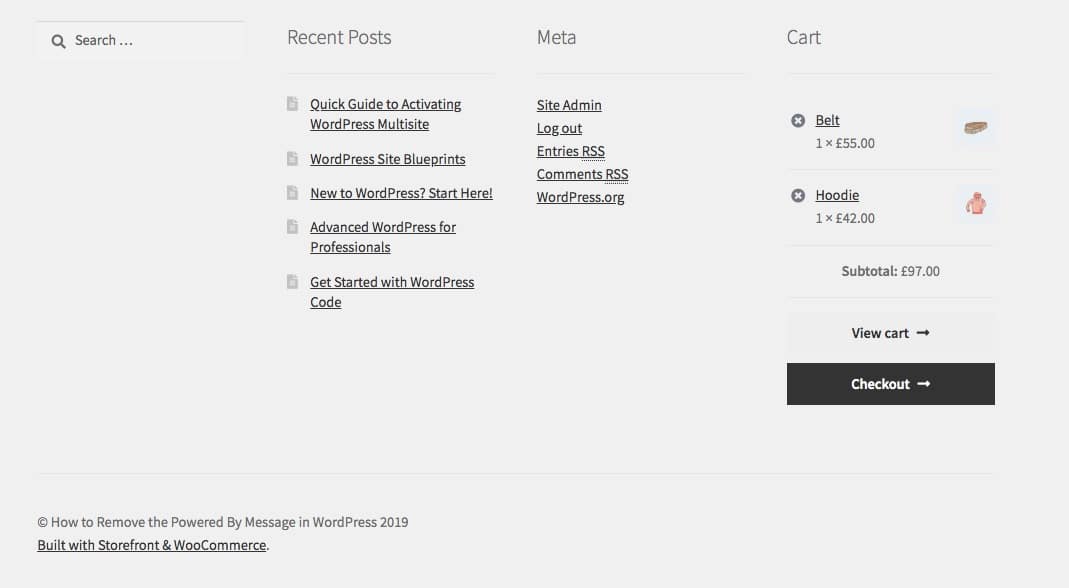A screen capture of a webpage's footer section showcases various functionalities and sections. On the far left is a search box, enabling users to search the website. The middle left column is titled "Recent Posts" and includes five navigational links to articles: "Quick Guide to Activating WordPress Multi-site," "WordPress Site Blueprints," "New to WordPress? Start Here," "Advanced WordPress for Professionals," and "Get Started with WordPress Code." 

Moving to the middle right column, titled "Meta," it features links for "Site Admin," "Log Out," "Entries RSS," "Comments RSS," and "WordPress.org." On the far right, the "Cart" section lists two items currently in the shopping cart: a belt priced at £55 and a hoodie priced at £42, bringing the subtotal to £97. Below the cart details are two buttons labeled "View Cart" and "Checkout."

At the bottom of the footer, a smaller section includes a copyright notice with the text "How to Remove the Powered By Message in WordPress 2019." Below this is a link indicating the site is "Built with Storefront and WooCommerce."